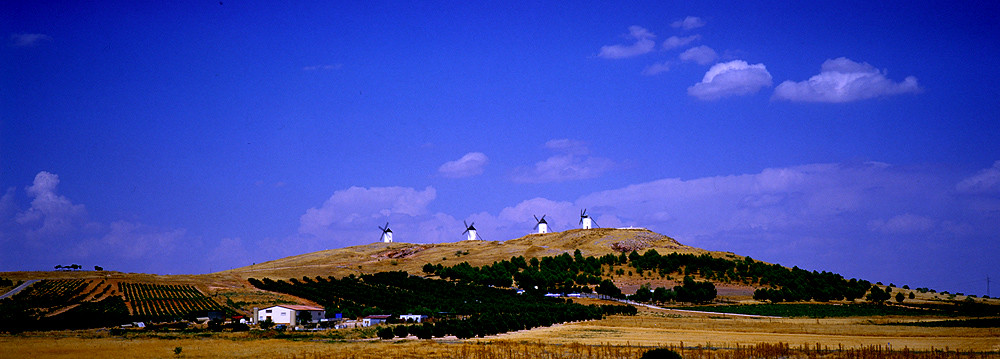The image depicts a wide and expansive outdoor scene with a stunningly blue, potentially edited sky making up about 70% of the frame and adorned with scattered puffy white clouds. Below the vibrant sky, a series of golden-yellow fields stretch across the bottom 30% of the image, interspersed with dark green trees that appear in a square formation, possibly indicating a tree farm. Dominating the horizon atop a brown hill, which slopes downwards to the foreground, are four windmills with white bases and dark-colored blades. They appear distant and small, emphasizing the vastness of the landscape. In the valley beneath these windmills, a white building and several smaller structures can be seen, while off to the left in the background, there are indistinct animals milling about, adding a touch of life to the serene and beautifully lit scene.